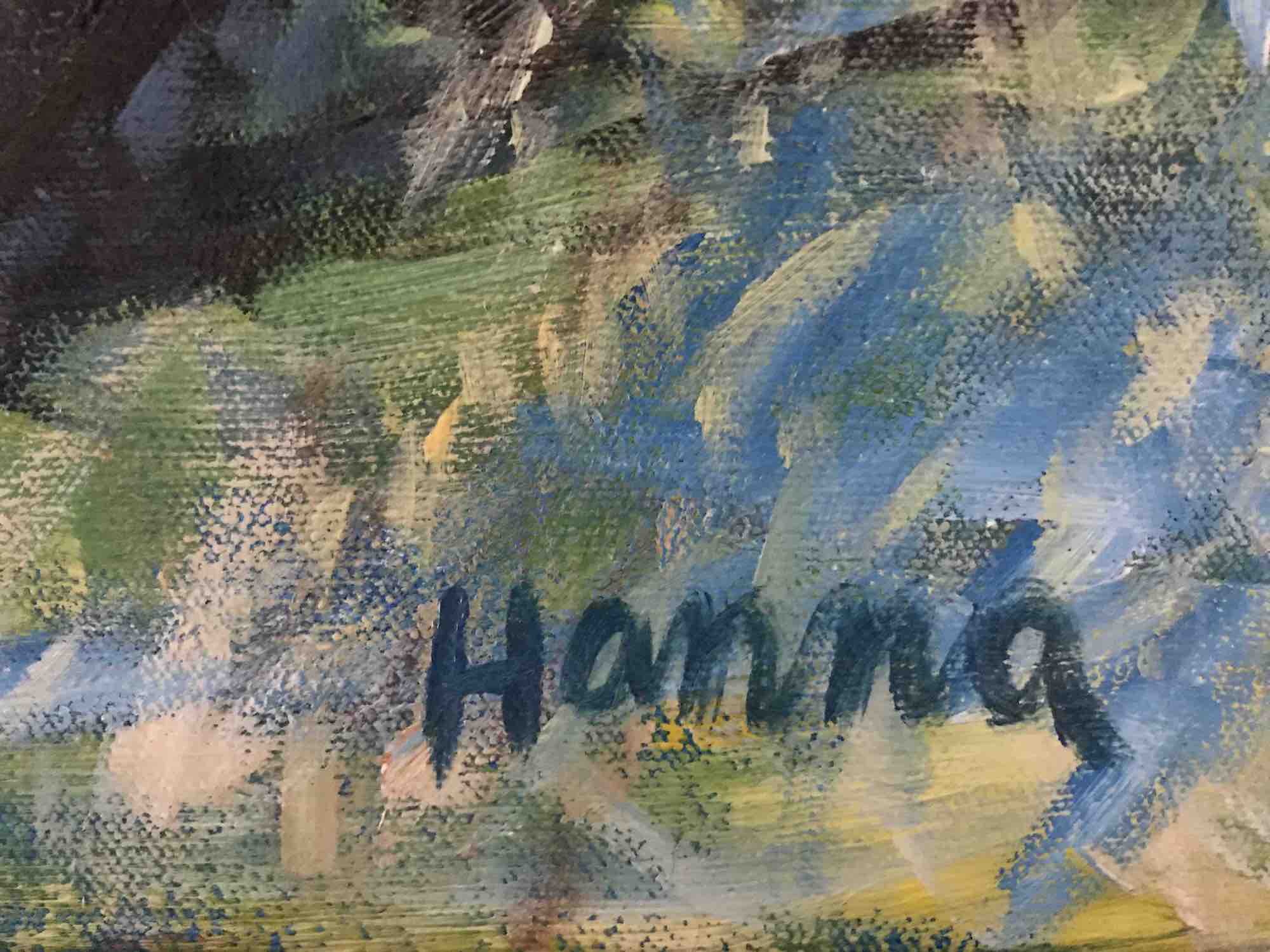This image features an abstract oil painting on canvas, characterized by the visible texture of the canvas within the broad, sweeping brushstrokes. Predominantly dark tones start at the top left corner with dense blacks accented by white streaks. As the colors gradient downwards, green dominates, interspersed with sections of blue. Near the center and extending towards the bottom right, the painting lightens into hues of light green, beige-white, and light blue, with hints of darker green specks, and eventually transitions into yellow. Some viewers might perceive the strokes as forming a vague, cloudy day or stormy atmosphere. The bottom right corner prominently features the signature 'Hannah' in a large-sized, cursive font, written in a dark green-blue paint. The signature is a standout feature, the first element that catches the eye in this zoomed-in view of the painting's lower section, framed by its abstract backdrop that may suggest a cliffside against water if viewed imaginatively.